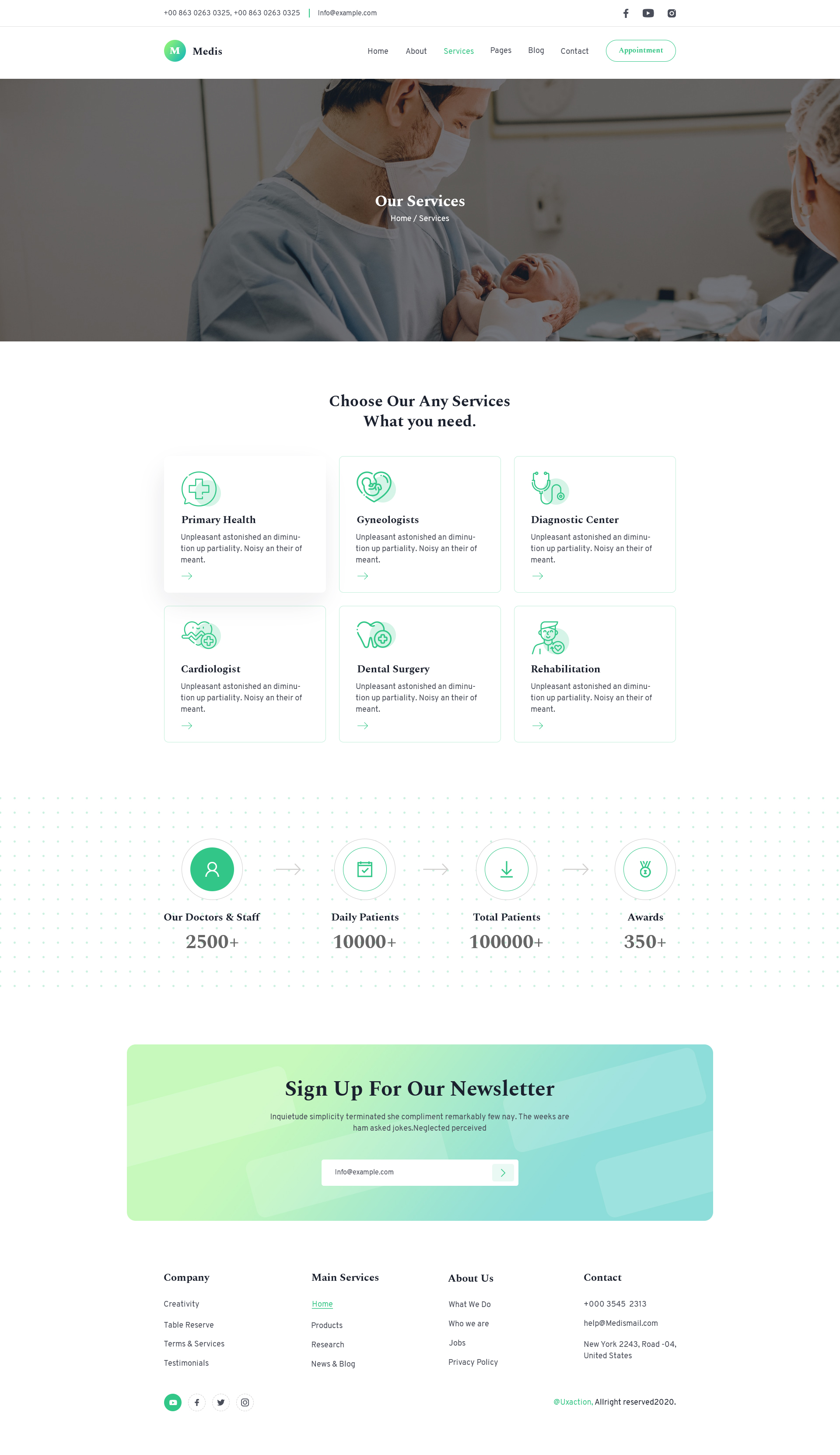In this somewhat blurry screenshot set against a white background, the focal point is in the upper left corner, where a white "M" sits within a green circle. To the right of this logo, the text reads "media" or possibly "medis." Below this header, a poignant photo captures a man clad in scrubs and wearing a white surgical mask. He gently cradles a newborn baby, whose mouth is wide open in a cry, swaddled securely in a white blanket.

Overlaying the image, a section titled "Our Services" is prominently displayed in bold white text, followed by a path indicator: "Home / Services." Beneath this text, a subheading instructs, "Choose any services you need."

Moving left to right, three white boxes are arranged, each labeled with a service and accompanied by a corresponding green icon:
1. "Primary Health" 
2. "Gynecologist"
3. "Diagnostic Center"

Below these options, the word "Cardiologist" appears next to a small green heart illustration. To its right, the text "Dental Surgery" is paired with an icon of a tooth, and finally, the word "Rehabilitation" is presented, suggesting a variety of medical services offered.